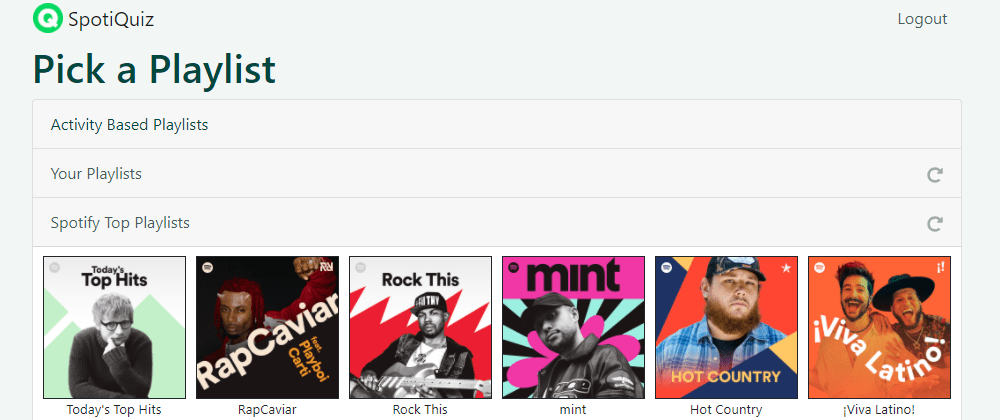The image is a wide rectangular graphic with a gray background. In the top left corner, there is a small green circle featuring a white letter "Q". Adjacent to it, the text "Spotty Quiz" is prominently displayed. In the top right corner, "Log Out" is written in black text.

Below "Spotty Quiz", there is a large, bold headline in black lettering that reads "Pick a Playlist", which is the most prominent text on the page. Underneath this, the categories "Activity-Based Playlists", "Your Playlists" (with a right-facing arrow in a circle), and "Spotify Top Playlists" (with another right-facing arrow in a circle) are listed.

The main section features six album covers arranged horizontally:
1. "Today's Top Hits" - Shows a man wearing glasses and a sweater, facing the camera.
2. "Rap Caviar" - A dark image featuring a person, with the text "Featuring Playboi Carti".
3. "Rock This" - Displays a man in a baseball cap holding a guitar.
4. "Mint" - Features another man in a baseball cap wearing a jacket.
5. "Hot Country" - Shows a bearded man in a blue checkered shirt wearing a baseball cap.
6. "Viva Latino" - Two men with open-mouthed smiles, one of whom wears a broad-brimmed hat, looking directly at the camera.